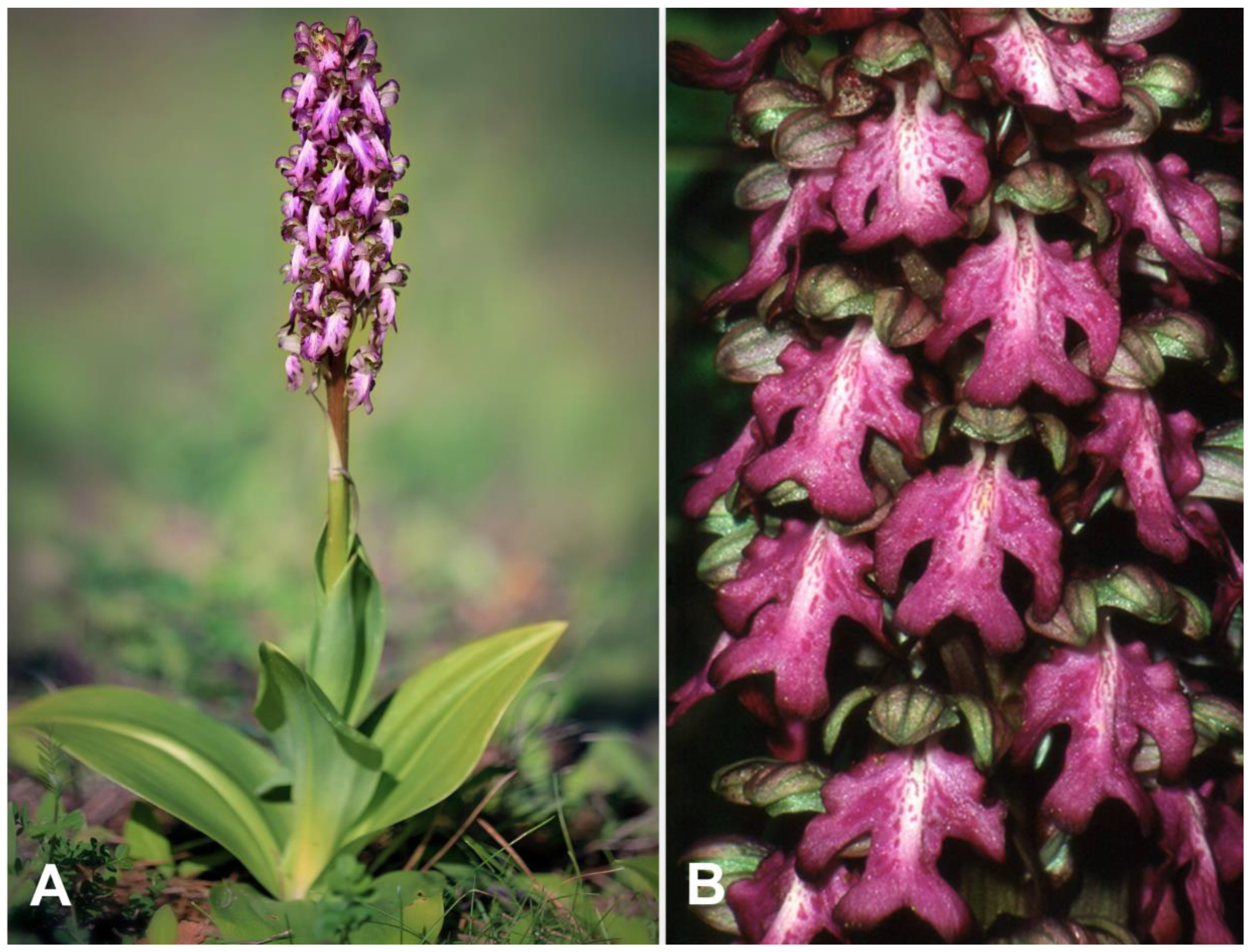In this set of two images labeled "A" and "B," we observe detailed shots of a flowering plant. Image A, on the left, captures the entire plant. It features a tall green stem, with green leaves near the base and small, budding pink flowers at the top. The background is softly blurred, hinting at a lush green environment, possibly a forest. The flowers at the top of the plant have pink petals with touches of white and darker edges, appearing almost purple or black. 

To the right, Image B offers an up-close view, concentrating on the intricate details of the flower petals. Here, the pink petals of the flowers are seen more clearly, showing white stripes down the middle and darker, almost purple edges. The background in this image is also blurred, further emphasizing the delicate, somewhat moist texture of the petals. This two-part illustration provides a comprehensive look at the plant, portraying both its full structure and the detailed beauty of its blossoms.